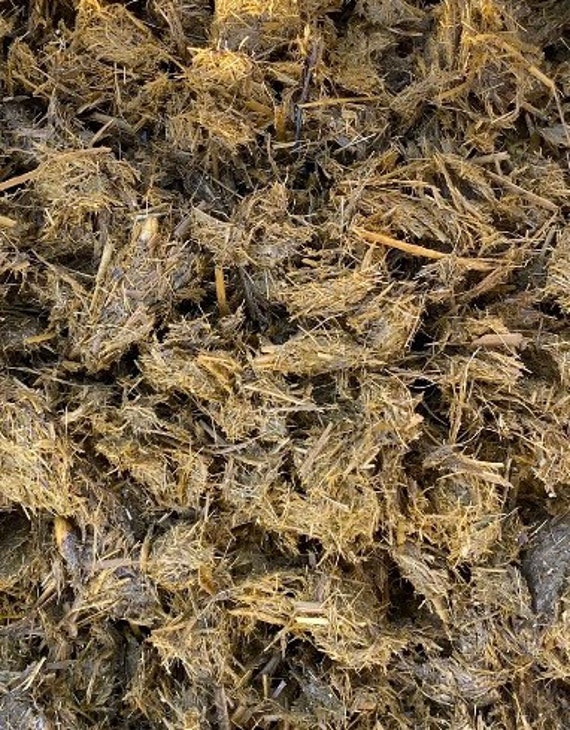This picture is a detailed, close-up shot taken from an overhead perspective of a clumped, interwoven mass of straw-like, yellowish-brown grass or hay. The portrait layout of the image emphasizes the texture of numerous clusters of this grass, some appearing dark and damp as if recently mowed or exposed to moisture. Interspersed among the grass are twigs and sticks that contribute to an overall earthy, nest-like appearance. The entire scene is devoid of any people, animals, text, or vibrant colors, relying solely on the natural palette of brown and tan hues. The top of the image seems slightly brighter, suggesting there is extra light hitting that particular section.